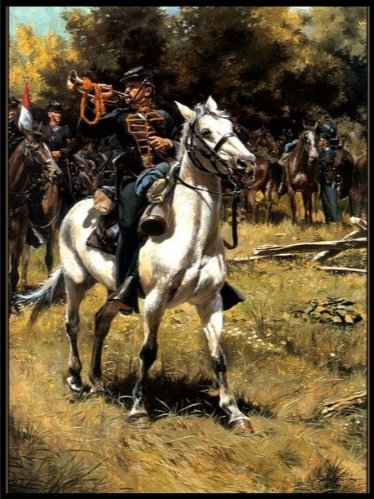The painting depicts a dynamic cavalry scene, likely set during the American Revolution or Civil War. At its center, a soldier in a dark blue uniform intricately detailed with gold braid sits astride a robust white horse, its head slightly cocked and raised upward. The soldier is blowing a bugle adorned with an orange string, possibly signaling to the men behind him. These men, some mounted and some standing, are amidst a field of trampled brownish-green grass interspersed with wildflowers and the remnants of a fallen tree trunk.

One notable figure directly behind the bugler carries a red and white flag, red on top and white on the bottom, though its exact significance is vague. To the right, a man stands beside a saddled horse equipped with military supplies. The background is richly detailed with a lush, green forest that has patches of yellow leaves and sparse glimpses of a blue sky peeking through. The overall composition suggests a sense of movement and urgency, capturing a moment of organization and readiness within the wartime landscape.